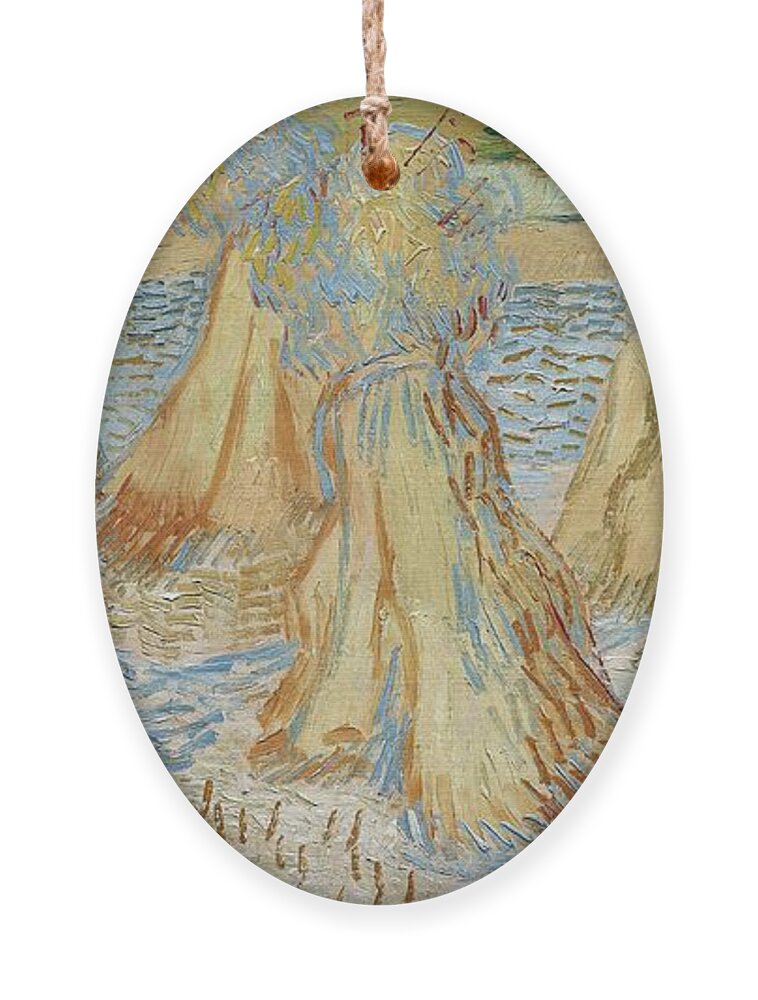The image showcases a small, oval-shaped pendant, intricately designed and apparently crafted from a thin piece of metal. Attached to the pendant is a piece of pinkish thread or rope, indicating it can be worn as a necklace. The pendant itself features an oil painting, depicting a volcanic landscape with steep, towering volcanoes. These volcanoes, numbering two or three, are brown with hints of blue and brown downward lines, suggesting an eruption scene with clouds of smoke in bluish, greenish, and whitish hues. Surrounding the volcanoes is a body of water, reflected through blue lines that represent waves. The painting style is impressionistic, rendering the scene in a way that evokes an ancient, almost mystical artifact.